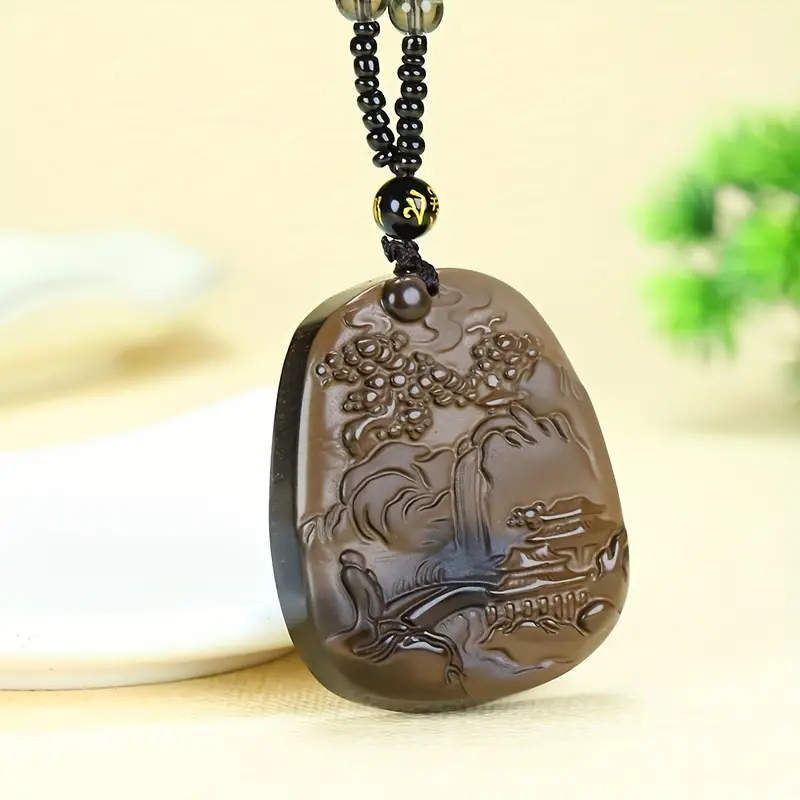This landscape-oriented color photograph showcases a pendant necklace as its central subject, slightly towards the bottom. The pendant is a rounded rectangle shape, primarily brown with a shiny, chocolate-like appearance, and features an intricate relief carving. The scene depicted on the pendant includes mountains, a waterfall, trees, a bridge leading to two buildings, and a person possibly reclining on a rock. The upper part of the pendant is adorned with a black bead inscribed with golden Asian lettering, adding to its detailed craftsmanship. The necklace chain is constructed of small, shiny black seed beads, with two gray crystal beads at the top, partially cut off from the frame. The background of the image is a light yellow color, featuring a blurred green plant in the top right corner and a white, rounded platter on the left, creating a warm and inviting ambiance. Overall, the photograph employs a style of photographic representationalism and realism, focusing on product photography.